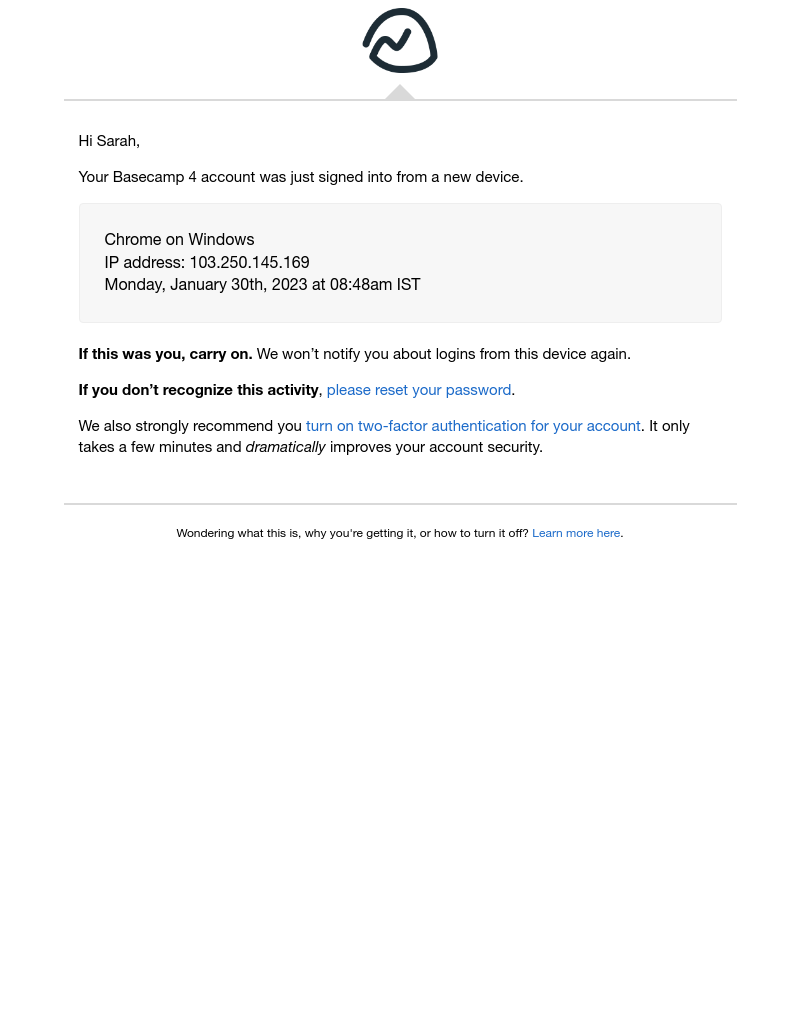A screenshot of an email notification with a crisp, white background. At the top, a black logo resembling a stylized 'D' is positioned above a thin gray line. Below the line, the body of the email is displayed in black font. The message begins with a greeting: "Hi Sarah," followed by an alert indicating that her Basecamp 4 account was accessed from a new device. 

Encased in a very light gray rectangle, the details of the login are provided: "Chrome on Windows, IP address: 103.250.145.169," followed by the timestamp: "Monday, January 30th, 2023, at 8:48 a.m. IST." 

The email continues to reassure Sarah: "If this was you, carry on; we won't notify you about logins from this device again." However, it also issues a caution: "If you don't recognize this activity, please reset your password," with "please reset your password" as a clickable blue link.

To further enhance security, the email recommends enabling two-factor authentication, highlighting that it "only takes a few minutes and dramatically improves your account security." The phrase "turn on two-factor" is also presented as a clickable link, inviting immediate action.